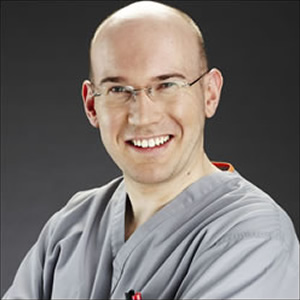This photograph appears to be a professional headshot of an unidentified white male, possibly intended for workplace use. He is predominantly bald, save for a slight fringe of dark hair above his ears, which is very closely cropped. The man is clad in a distinctive gray top, resembling scrubs, with a crossover front design. There is a hint of red on the collar at the back and a partially visible logo on the left side, which seems to feature a blue star and a red and white star, though the specifics are unclear.

His glasses are rimless, lending a subtlety to his facial features, with only the dark earpieces noticeable. The color of his eyes is indeterminable, though they appear to be light. He is captured in an amiable expression, smiling broadly to reveal his upper teeth. The background is a solid, very dark gray, and the frame of the image extends from just above the top of his head to just below his shoulders, including the upper part of his arms. Given his attire and appearance, he gives the impression of being either a physician or an astronaut.